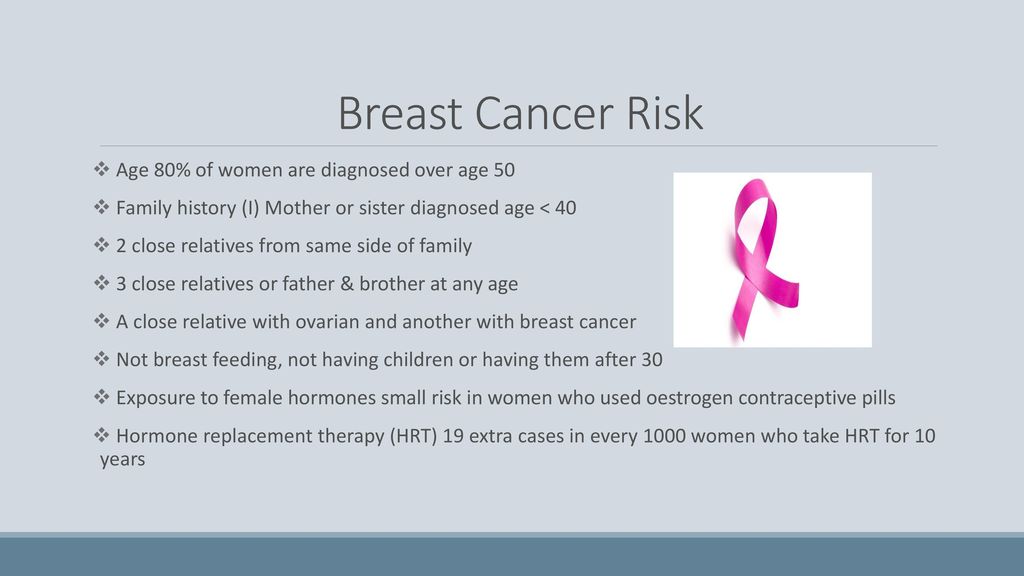[Image Description: The image has a gray background with the following information presented in black text.]

Title: Breast Cancer Risk Factors

1. **Age:**
   - 80% of women diagnosed are over age 50.

2. **Family History:**
   - Mother or sister diagnosed by age 40.
   - Two close relatives on the same side of the family.
   - Three close relatives, or a father and brother, diagnosed at any age.
   - A close relative with both ovarian and breast cancer.

3. **Reproductive History:**
   - Not breastfeeding.
   - Not having children or having them after age 30.

4. **Exposure to Female Hormones:**
   - Small risk associated with women who used estrogen contraceptive pills.
   - Hormone Replacement Therapy: 19 extra cases of breast cancer per 1,000 women who take HRT for 10 years.

To the right of the text, a pink ribbon, symbolizing breast cancer awareness, is displayed against a black and white background. The bottom edge of the image has a blue-green (or sea green) border.